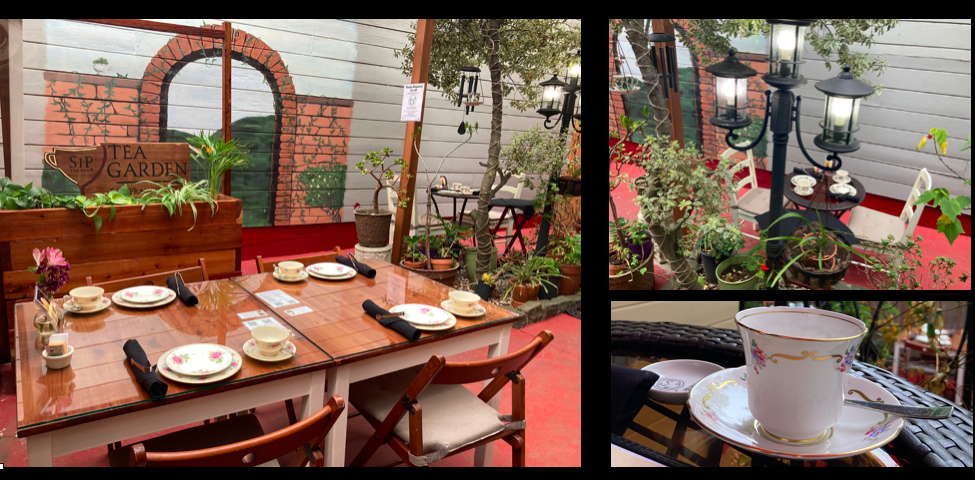This descriptive collage showcases an enchanting outdoor setting of the "Sip Tea Garden" cafe, meticulously spread across a landscape-oriented image consisting of three distinct photos with dark black borders. The largest section, dominating the left side, presents a serene outdoor dining area. Here, two wooden tables with glass overlays are set up with four white, cushioned, folding chairs. The tables are adorned with place settings, featuring floral plates, white mugs, black napkins bundled with silverware, and fresh flowers in vases. A wooden sign etched with "Sip Tea Garden" hangs in the background amidst an artistic mural depicting a brick archway, enhancing the rustic charm of the scene. The backdrop reveals lush greenery with trees and lanterns hanging, adding to the ambience.

The upper right photo centers on a vintage black street lamp, elegantly illuminating a small circular table paired with two white chairs beneath it. This area is surrounded by potted plants, blending seamlessly with the natural decor of the cafe. The bottom right photo provides a close-up view of a white coffee mug with a floral pattern, resting on a matching saucer with a silver spoon, placed on a glass tabletop, highlighting the attention to detail in the cafe’s presentation.

Together, these images capture the inviting and tranquil atmosphere of "Sip Tea Garden," where detailed decor and natural elements combine to create a perfect outdoor dining experience.